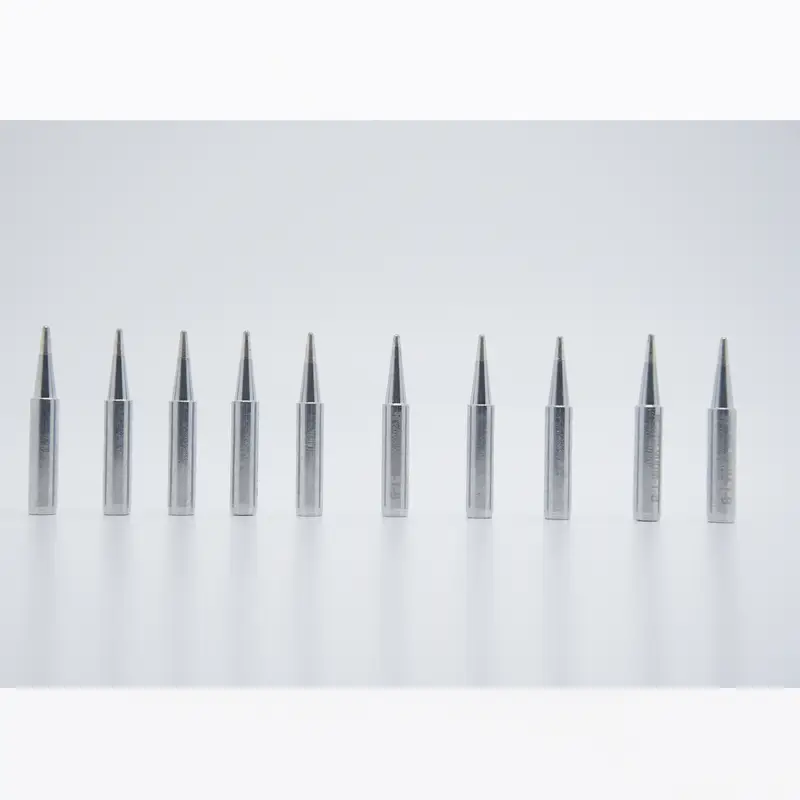In this image, a sleek, light gray background sets the stage for a meticulous arrangement of ten silver bullets. Positioned side by side with about an inch of space between each one, they form a precise, orderly line. The bullets are crafted with long cylindrical bodies that taper into exceptionally sharp points, reflecting a cool metallic sheen under the bright lighting. Shadows cast on the surface add depth and dimension, highlighting their polished finish and emphasizing their potential lethality. Despite the lack of specific firearm details, the sharpness and craftsmanship suggest they are designed for serious impact.